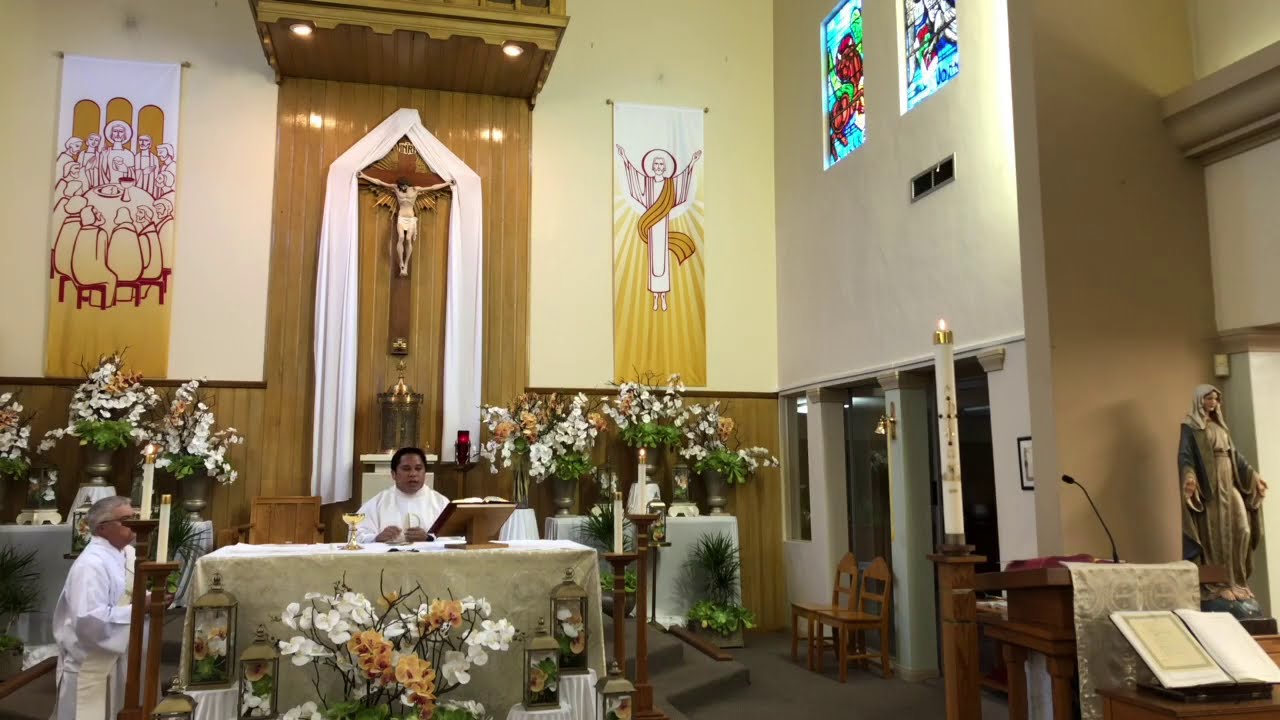The image depicts the serene interior of a church adorned with intricate details. Dominating the scene, a man clad in a white robe stands behind an altar covered with a cream-colored tablecloth, where an open Bible rests on a wooden book stand. To his right, another man in a similar white robe, this one older with grayish hair, stands near some wooden candle holders. 

The backdrop features a striking wooden cross with a figure of Jesus, arms outstretched, draped in a white sash. Flanking the cross are elegant banners: the left one portrays the Last Supper with people gathered around a table, and the right one shows a figure with raised arms, both set against a gold and white backdrop with intricate red outlining. Below these are several large vases brimming with white flowers, further adding to the ornate setting.

On the right-hand wall, two stunning stained glass windows with primarily red and blue designs capture the eye, adding a splash of vibrant color to the space. At the bottom of this wall is an open doorway, accompanied by two wooden chairs. A statue of the Virgin Mary, another Bible on a raised platform, and a pew with a microphone are also visible on the right side, adding to the richness of the scene. The combination of these elements—a harmonious blend of spiritual symbols, vibrant art, and solemn furnishing—captures the essence of this sacred space.